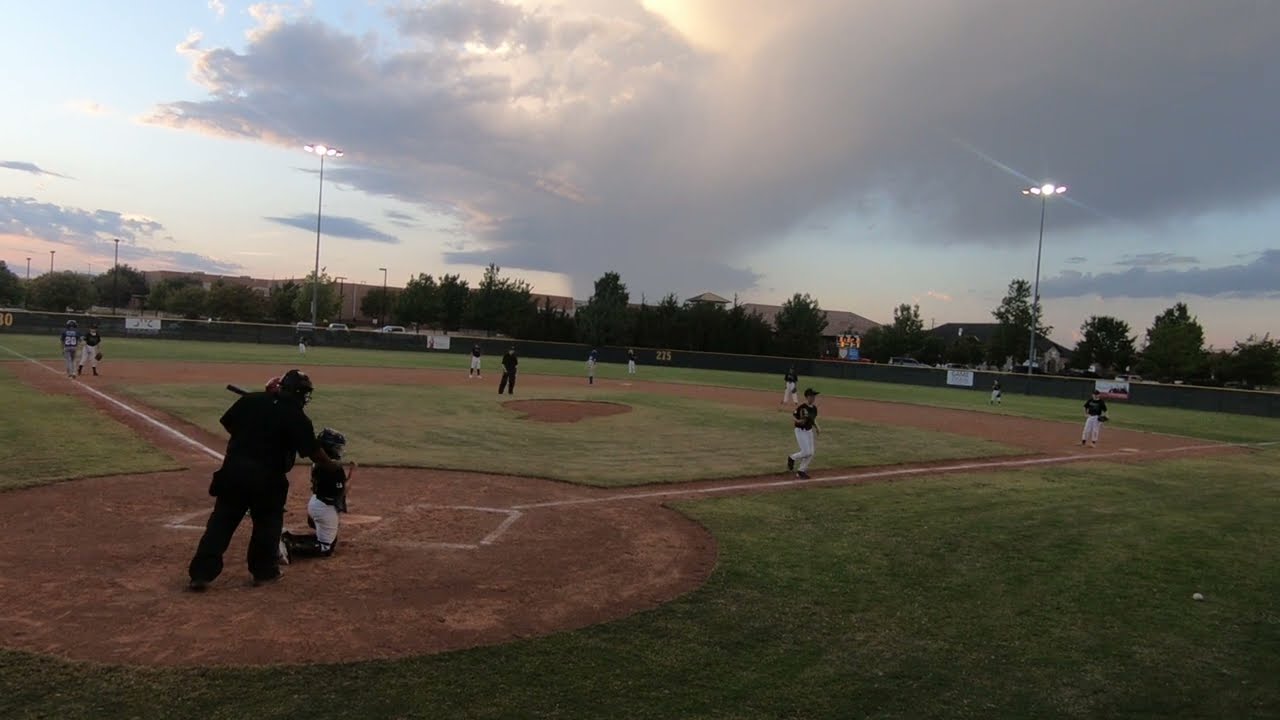The photograph captures a pivotal moment at a local baseball game around sunset. The sky is a blend of light blue and pinkish hues, partly obscured by a large, white, puffy cloud. The lighting is dim, with the stadium floodlights already turned on to illuminate the field as dusk approaches.

The image is taken from a vantage point slightly behind and to the right of home plate, providing a clear view of the action. In the lower-left portion, an umpire dressed in all black stands in the foreground, possibly handing a ball to the catcher kneeling behind home plate. The catcher, wearing a dark top, dark cap, and white pants, is ready to receive the pitch, aligning with the official nature of the game, suggested by the players' proper jerseys and white baseball pants.

On first base, a runner dashes towards the base, while another figure stands poised on third base. The pitcher's mound is vacant, with a player dressed similarly to the umpire crossing the baseline, though not standing on the mound.

The infield's clay baselines and batter circle are sharply delineated with white chalk, transitioning into the grassy outfield. Surrounding the field, a chain-link fence features scattered advertisements and distance markers. Trees line the background beyond the fence, adding to the picturesque scene. The floodlights atop tall poles are prominently lit, ensuring the game continues as evening sets in.